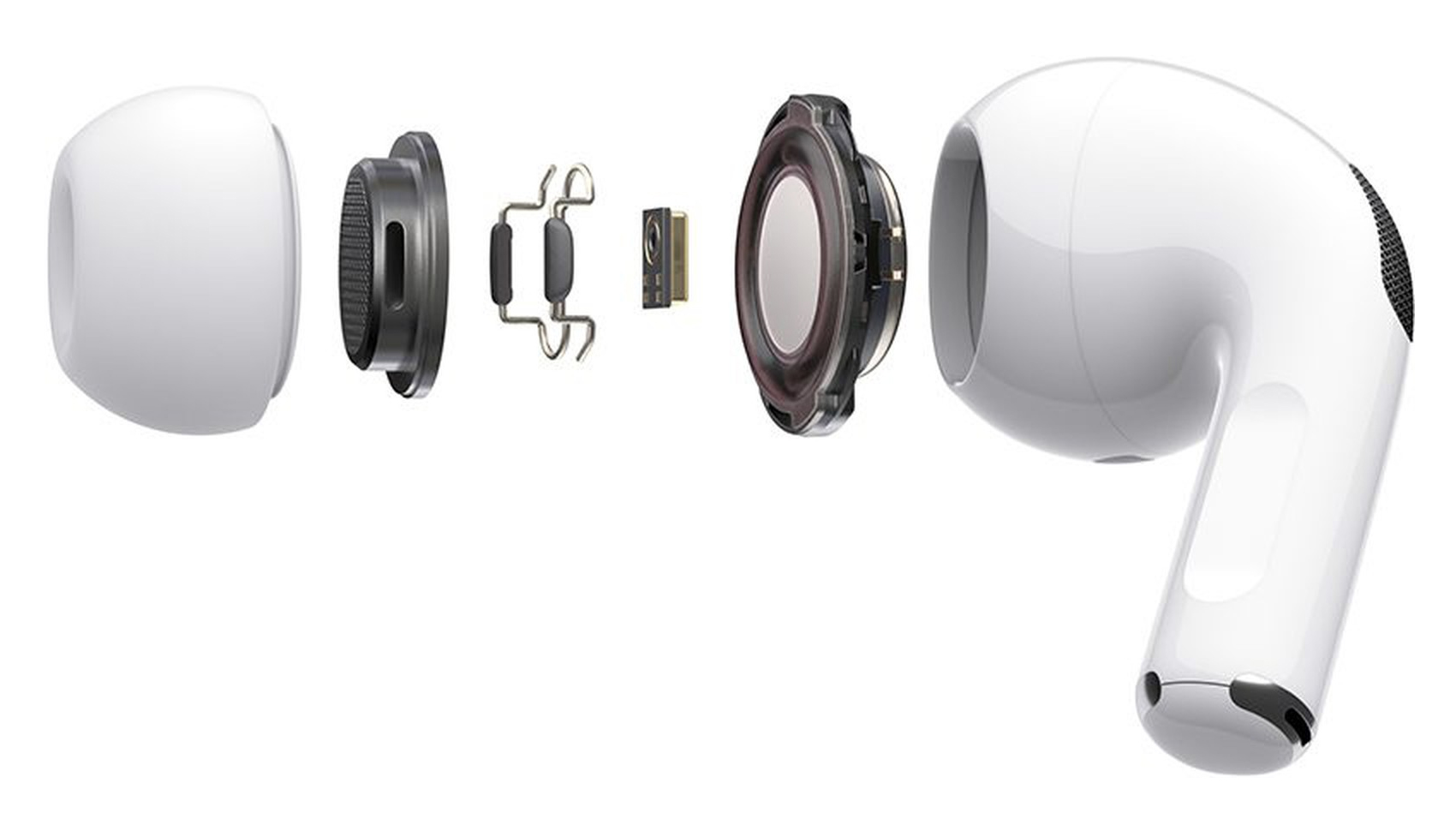The image is a staged, full-color photograph with a horizontally rectangular orientation and no border, set against a pure white background, devoid of any text or living elements. It features a disassembled wireless earbud displayed in a detailed, schematic-like fashion. The main body of the earbud, positioned on the far right, is predominantly white with a bit of black and silver detailing where the earbud's "head" meets its "stem." To its left lies a series of intricately arranged components showing the internal parts of the device. The first component looks like a button or the face of a watch without the wristbands, likely representing the actual speaker part. Next to it, there are several metal pieces including a rectangular one and a couple of bent wires, demonstrating the intricate inner workings. Further to the left, additional parts such as another cap-like piece and the outer earbud casing are laid out, illustrating the different layers and assembly of the earbud.